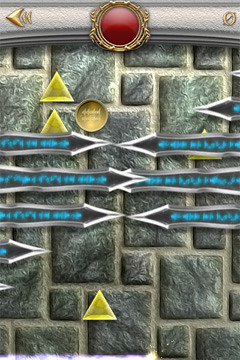Here is a cleaned-up and detailed caption for the image:

---

*Screenshot from 'Hand of Greed' Video Game*

The image depicts a screenshot from the video game "Hand of Greed." The top portion of the screen features a horizontal gray bar that spans the entire width. Within this bar, there is a gold right-facing arrow on the right-hand side, presumably serving as a back or forward navigation button. At the center of the bar, a prominent round red jewel, resembling a ruby, is encased in an ornate gold filigree frame. To the left of the jewel, a gold zero with a diagonal line through it is visible.

Beneath the gray bar, the background consists of a pattern of gray stone blocks of varying sizes, arranged without a specific order. The scene includes three noticeable yellow triangles. Two of these triangles are positioned near the top right side, aligned vertically, one directly below the other. The third triangle is located slightly right of center at the bottom of the screen. 

An additional gold circle is present to the left of the upper two triangles. Intersecting lines, designed as arrows, traverse the screen horizontally in three rows. These black lines, highlighted with blue shading, create intersections where the arrow tips meet or overlap. At the top left and bottom right corners of the screen, two arrow tips are visible: one pointing left and one pointing right, respectively.

The overall composition of the screen elements suggests a tactical or puzzle-like interface, featuring navigation, indicators, and possibly strategic components within the game's environment.